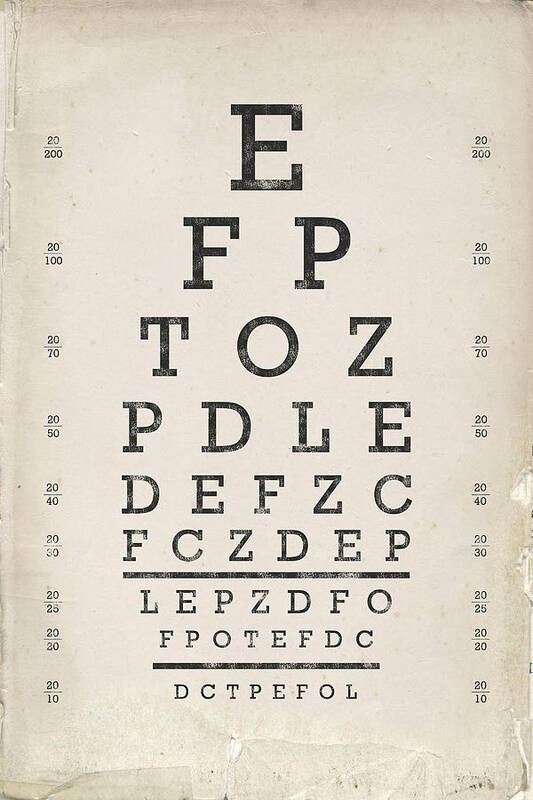This image depicts an eye doctor's wall chart, characterized by its vertical rectangular shape and light gray background, showing signs of age with weathered and slightly tattered or wrinkled edges. The chart, used to test visual acuity, features rows of letters that progressively decrease in size from top to bottom, starting with a bold uppercase "E." The lines below the topmost letter diminish in size, with the smallest letters still being fairly readable, suggesting the chart must be positioned at a considerable distance from the observer.

Accompanying each row of letters on both the left and right sides of the chart are fractional numbers indicating the vision quality of an individual able to read each specific line. These numbers start from "20/200" at the top and decrease through "20/100," "20/70," "20/50," "20/40," "20/30," "20/25," "20/20," and finally "20/10" towards the bottom. 

The center column of the chart lists the letters in descending size as follows: "E," "FP," "DOZ," "PDLE," "DELZC," "FCZGEP," an undefined black underline, "LEPZBFO," "FPOTEFDC," another black underline, and finally "DCTPEFOL."